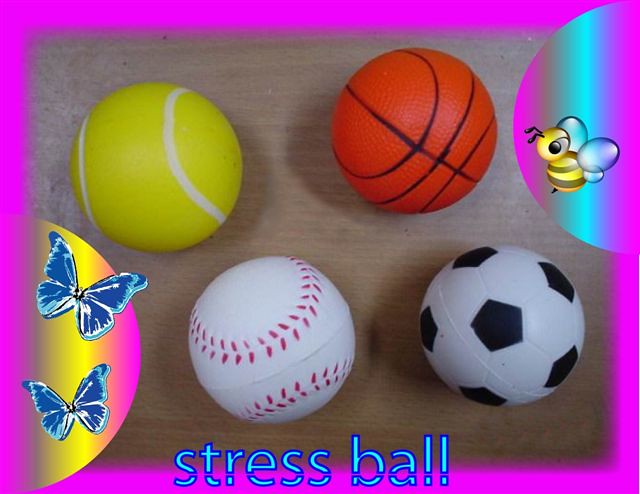The promotional image features a collection of four stress balls, each styled to resemble different sports balls. The stress balls, arranged on a light oak-colored table, include a tennis ball (top left), a basketball (top right), a baseball (bottom left), and a soccer ball (bottom right). The image has a distinctly vibrant, digital frame with a glowing neon pink border. At the top right, a semicircular tab extends into the frame, showcasing a bright yellow and black 3D-rendered bumblebee with translucent aqua wings. Similarly, another semicircular tab at the bottom left features two blue butterflies with white and aqua accents on neon yellow and pink background. The bold, glowing text "Stress Ball" runs along the bottom edge of the frame, highlighting the nature of the product.